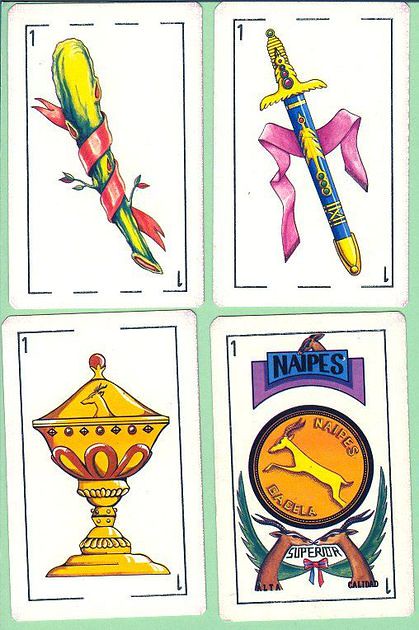The image showcases an animated or graphic depiction of four distinct playing cards. Each card is unique and intricately designed, contributing to an overall theme of fantasy elements.

1. The top left card features a black border. The number "1" is prominently displayed in both the top left and bottom right corners. At the center of this card is a piece of cactus adorned with a red ribbon wrapped around it.
   
2. The bottom left card displays a golden chalice with an intricately carved reindeer adorning its top. This card also bears the number "1" on it.

3. On the bottom right card, the heading reads "N.A.I.P.S." At the center lies a gold coin, embossed with an artistic depiction of a deer or similar animal. Additionally, two smaller deer figures are positioned at the bottom of the coin.

4. The top right card presents a striking blue dagger with a pink ribbon draped behind it and a gold hilt, completing the set with an intriguing contrast.

Each card in this collection is meticulously designed, showcasing a blend of natural and mythical symbols with elegant details.